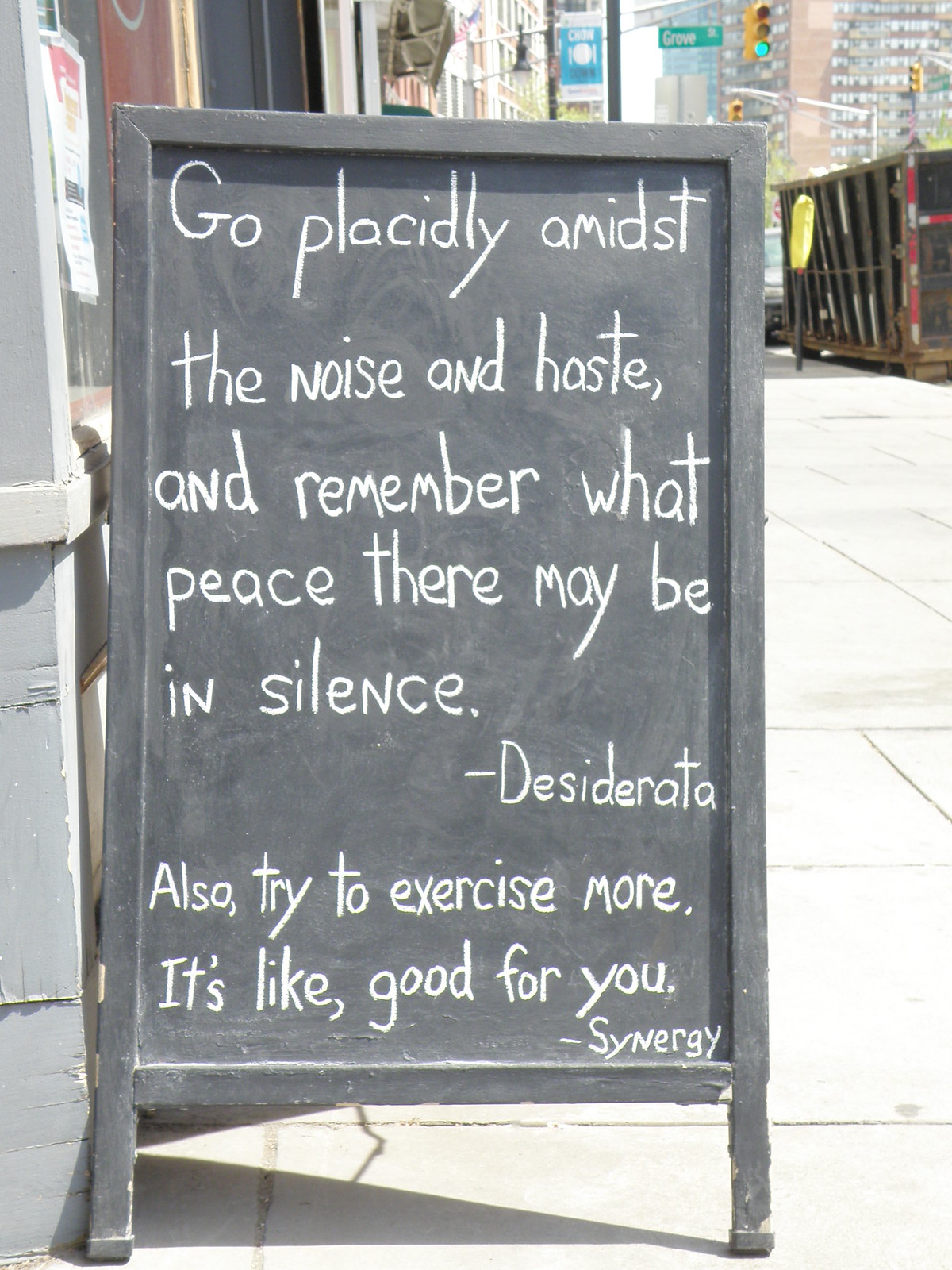The photograph captures a chalkboard easel placed on a gray concrete sidewalk in a bustling cityscape, potentially New York, Chicago, or even Toronto. The chalkboard, written in white chalk, displays the words:

"Go placidly amidst the noise and haste, and remember what peace there may be in silence. Desiderata. Also, try to exercise more; it's like good for you. Synergy."

In the background, tall buildings, a green traffic light, and a large dumpster are visible, along with a street sign for "Grove Street." The city ambiance, complete with sidewalks and apartments, suggests a vibrant urban setting where the chalkboard likely serves as an eye-catching advertisement for a business named Synergy.